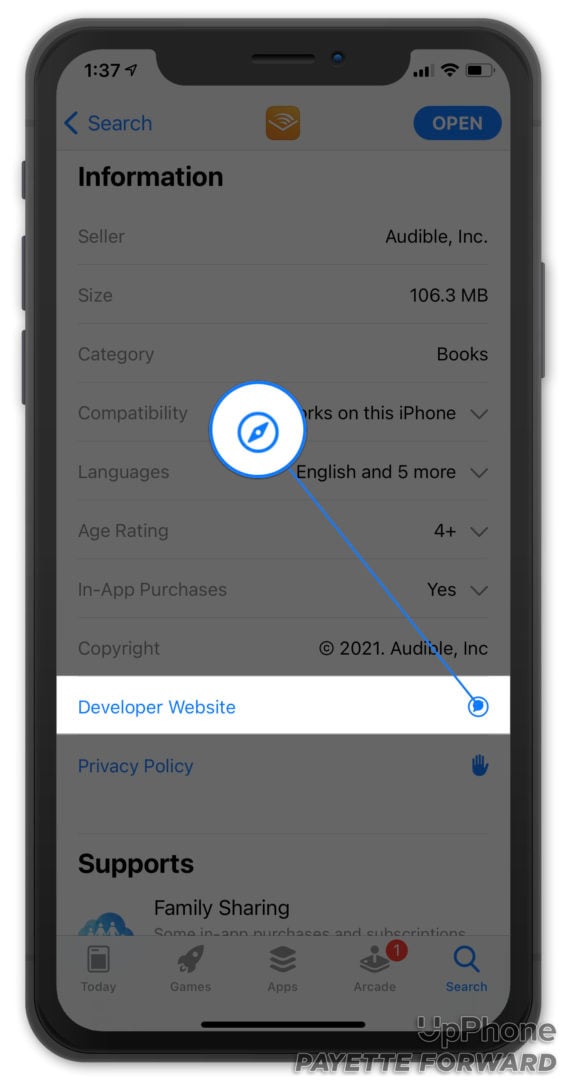The image displays the screen of a smartphone with various elements related to an app purchase. In the lower right corner, there's a logo displaying the text "UP Phone Payette Forward," though it is slightly garbled. The primary content on the screen details an app, with the seller listed as Audible Inc. The app size is noted as 106 MB and falls under the books category. It is compatible with the given phone and supports English along with five other languages. The app has an age rating of 4+ and includes in-app purchases. Copyright information at the bottom credits Audible Inc, with the year 2021.

Central on the screen, white-highlighted text reads "Developer Website," while other elements, including "Privacy Policy," appear grayed out. There is a notable graphic with a white circle and a blue line connecting it to an icon on the right side of "Developer Website," although its purpose is unclear.

At the bottom of the screen, navigation options are visible, including "Today," "Games," "Apps," "Arcade," and "Search." The entire screen and its details convey a user's interaction with an app page, possibly within an app store or similar platform.